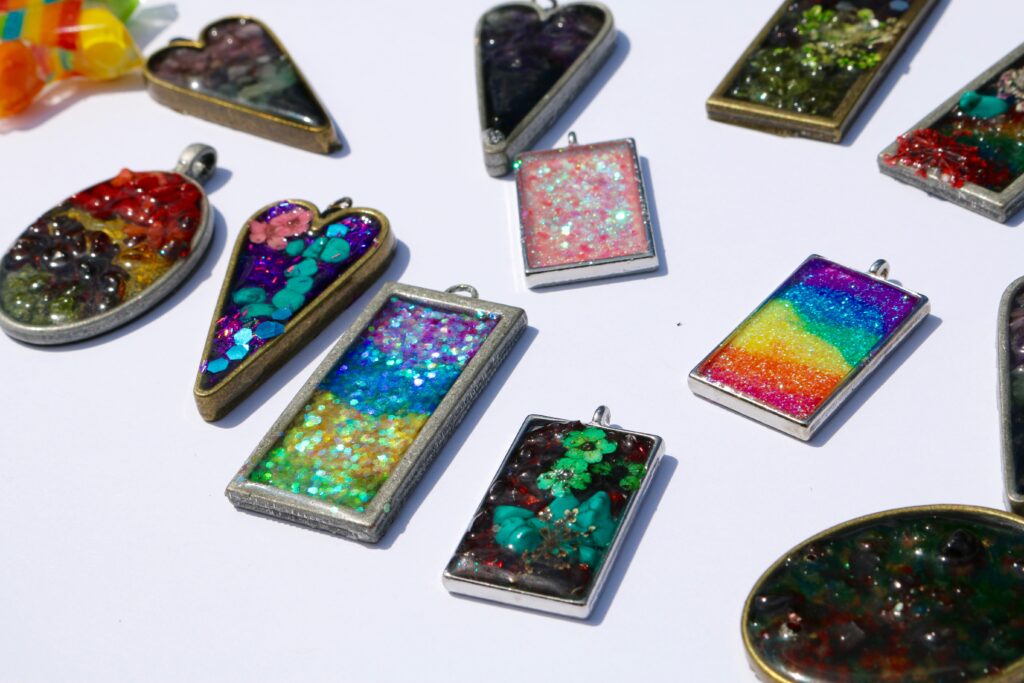A collection of 15 colorful and glittering pendants, varying in shapes—rectangular, oval, and heart-shaped—are displayed on a white surface. Each pendant features a small hook at the top, designed to connect to a chain or string, as they have no chains attached. The pendants are adorned with beads and intricate, glittery designs in an array of colors, such as pink, orange, yellow, green, blue, purple, and black. Notably, one rectangular pendant showcases a vibrant, rainbow-colored pattern, another heart-shaped pendant is plain, while another heart-shaped one has a sleek black lacquer finish. A small bowl filled with colorful beads sits at the bottom right corner, possibly for further decorating these ornate pieces.